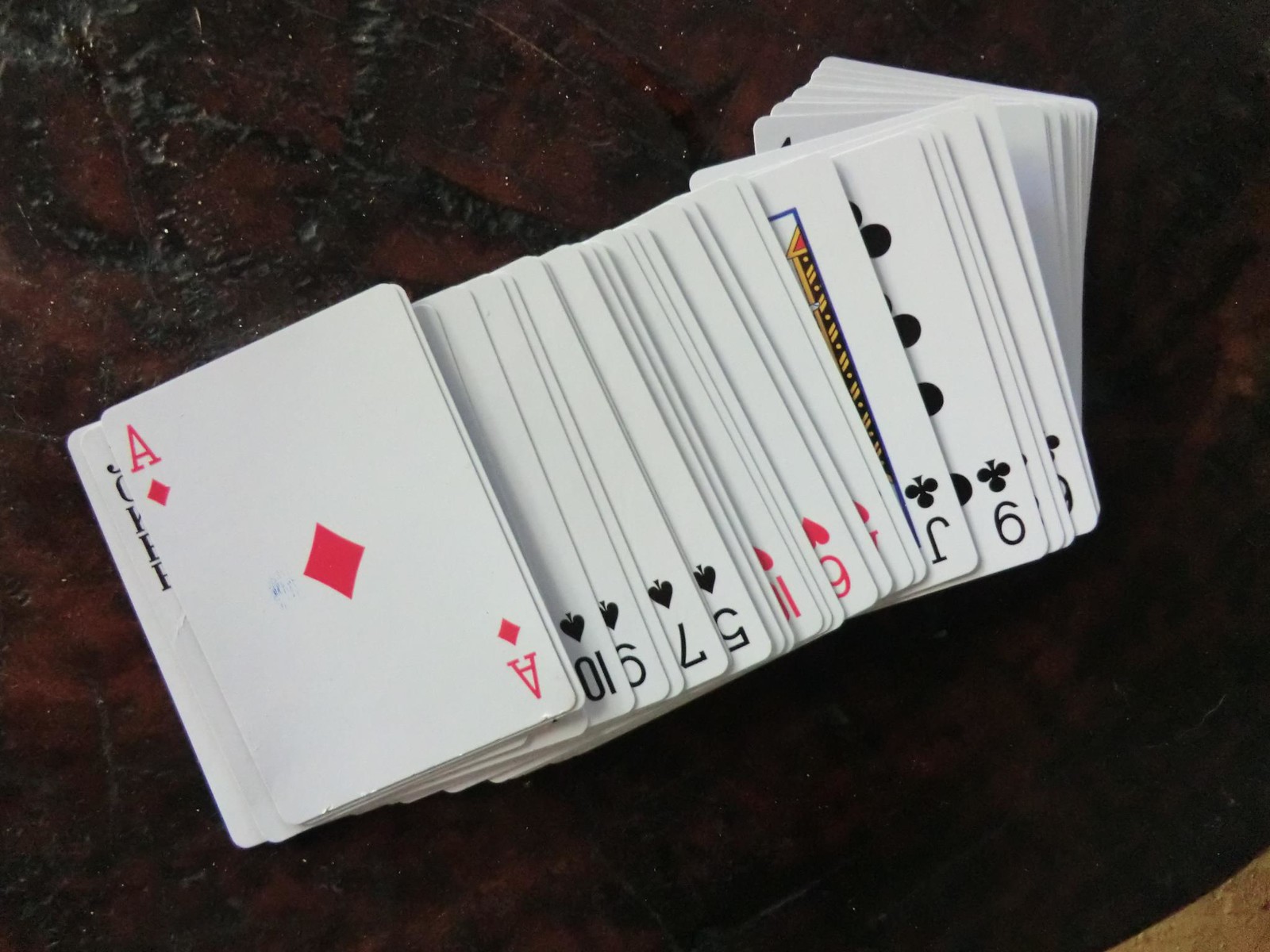This image captures a horizontal, rectangular photograph of a deck of playing cards, arranged in a fanned-out display. The prominent card is the Ace of Diamonds, positioned at an angle such that its top edge points towards the upper left corner of the frame, while the bottom edge faces the center of the bottom edge. The Ace of Diamonds, a pristine white card, features a red diamond in its center and matching red 'A's in the top left and bottom right corners, with the latter 'A' appearing upside-down.

Peeking out from beneath the Ace of Diamonds is a partial glimpse of a Joker card, identified by small sections of black lettering spelling "JOKER." To the right of the Ace, the remaining deck is splayed out, showcasing several cards in a variety of suits. In order of visibility, there are the 10 of Spades, 9 of Spades, 7 of Spades, and 5 of Spades, all in black and appearing upside down, creating a visually intriguing spread.

Further along, a hint of a red heart is visible, followed by another card bearing a red 6 of Hearts. In the ensuing cards, only partial segments, including a red dot and another half-heart, can be seen, suggesting the presence of several stacked cards. Additionally, an upside-down Jack of Clubs makes an appearance, distinguished by the visible 'J' and clover motif. Another card with a black 9 of Clubs also displays prominently, adding to the array.

The fan of cards rests atop a richly colored, brownish-red surface, accented by black streaks and a touch of tan in the bottom right corner, providing a warm and textured backdrop to the scene.